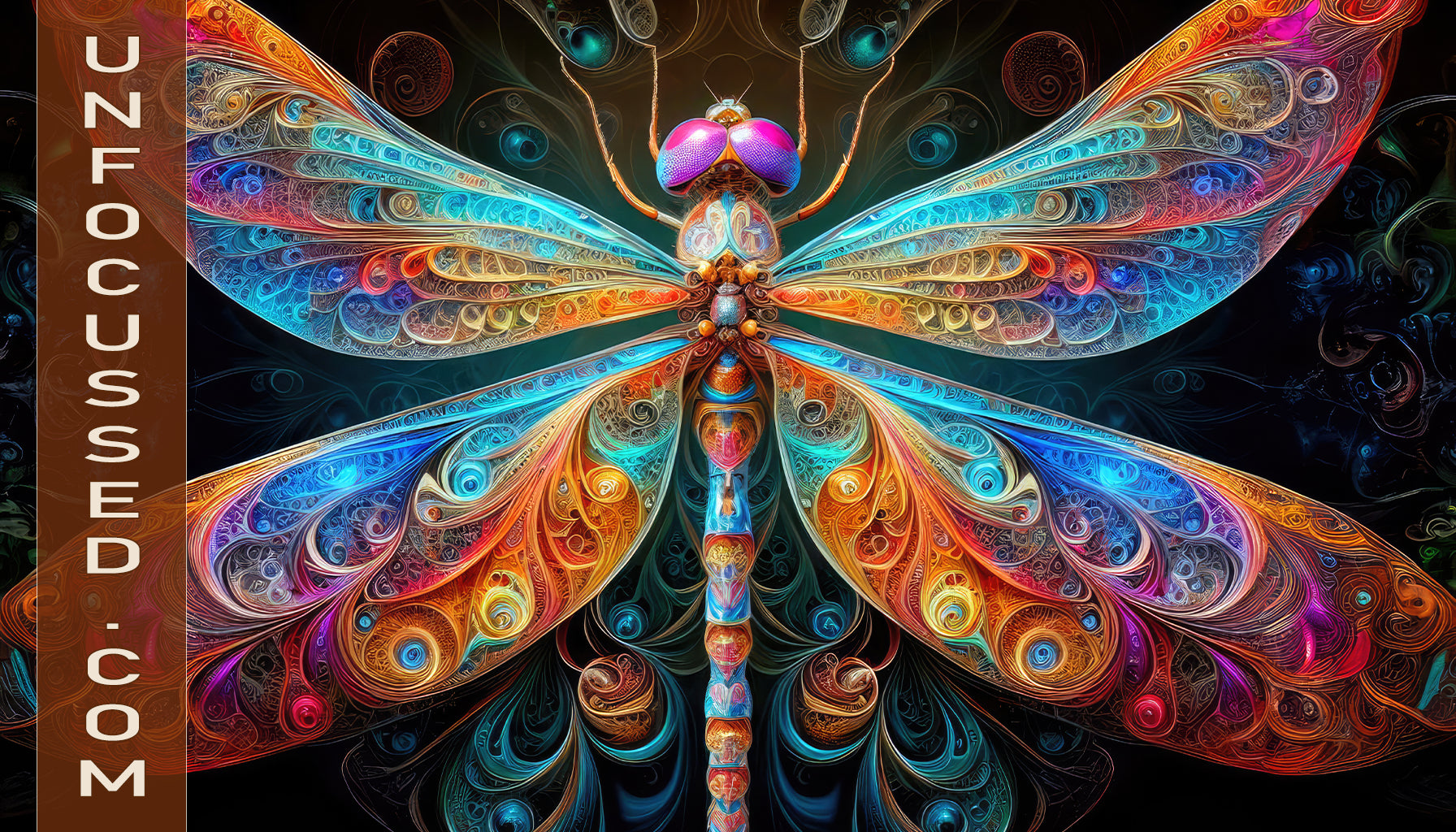The image features a prominently displayed vertical banner on the left-hand side with the text "unfocused.com" written in white. The main subject of the image is a stunning, colorful digital portrait of a dragonfly. This psychedelic artwork showcases the dragonfly with four teardrop-shaped wings, vividly patterned with a myriad of colors including blues, reds, yellows, pinks, oranges, and purples. Each wing features intricate, peacock-like swirls of color. The dragonfly's segmented body is long and narrow, stretching almost from the top to the bottom of the image. Its eyes are particularly striking, rendered in pink and purple hues. The background complements the dragonfly with its own swirling, psychedelic patterns in blue and orange, adding to the vibrant and mesmerizing aesthetic of the overall image.